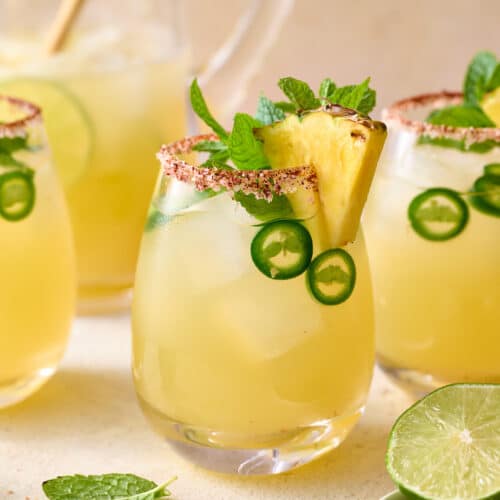The photograph showcases a meticulously arranged setup of three identical oval-shaped glasses filled with a vibrant yellow liquid, identified as a potential cocktail. Each glass contains three square ice cubes, thin slices of jalapenos, fresh mint leaves, and is garnished with a triangular wedge of pineapple perched on the salt-rimmed edge. The rims are coated with a distinctly brown salt, adding a touch of sophistication.

Positioned on a pristine flat white surface, the scene is complemented by a single mint leaf near the left corner and a halved lime at the bottom right. In the top left corner, a clear glass pitcher, half-full and containing lime slices and a large stirring utensil, stands ready. This visually enticing arrangement, with its evenly distributed soft lighting, reflects a high level of professional food photography skill, possibly even AI-generated in its perfection.